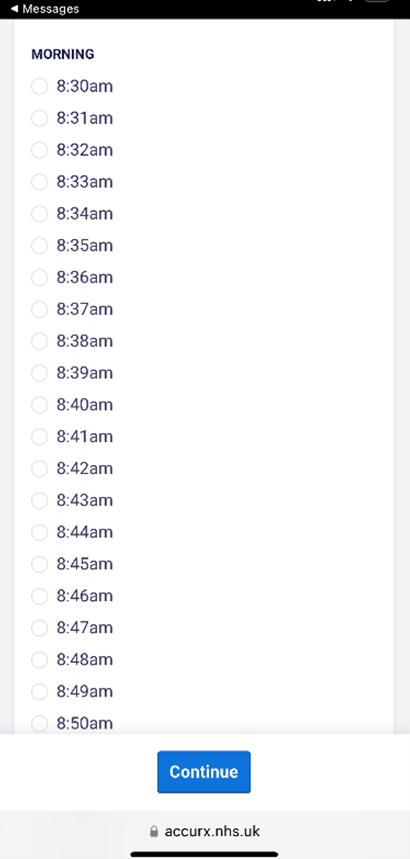In this image, we see a screenshot from a cell phone displaying a list of alarm times. At the very top left corner, the word "Messages" is displayed in white text against a black background. Directly below this, the heading "Morning" appears in black text.

Underneath the "Morning" header, there is a vertical list of alarm times, starting from 8:30 a.m. and increasing by one-minute intervals. The times listed are: 8:30 a.m., 8:31 a.m., 8:32 a.m., 8:33 a.m., 8:34 a.m., 8:35 a.m., 8:36 a.m., 8:37 a.m., 8:38 a.m., 8:39 a.m., 8:40 a.m., 8:41 a.m., 8:42 a.m., 8:43 a.m., 8:44 a.m., 8:45 a.m., 8:46 a.m., 8:47 a.m., 8:48 a.m., 8:49 a.m., and 8:50 a.m. Each time is followed by the abbreviation "a.m." printed on its right.

The list of times is set against a white background, while narrow, light gray vertical borders run along the left and right edges of the screen. At the bottom of the image, there is a blue "Continue" button, implying user interaction to proceed further.